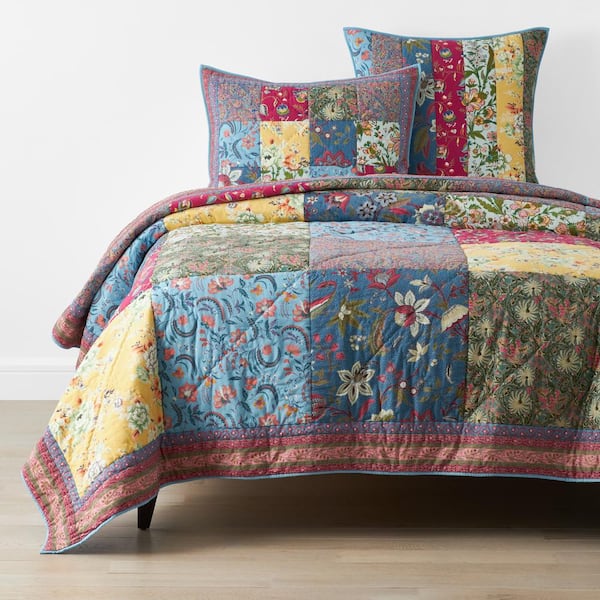This photograph captures a well-lit bedroom showcasing a beautifully adorned bed with a colorful quilt and matching pillows. The quilt is a vibrant patchwork featuring various fabric tiles stitched together, displaying an array of floral and leaf patterns in shades of light blue, dark blue, green, yellow, and red. The quilt is outlined with a red and pink banner-like edge. On the bed, there are two pillows; the one on the left mirrors the quilt's design with smaller tile patterns, while the one on the right features vertical stripes of the same colorful fabrics. The bed rests on a light brown wooden floor, and the backdrop is a light grey wall. The photograph is taken from the perspective of the foot of the bed at about mattress height and has a square format.